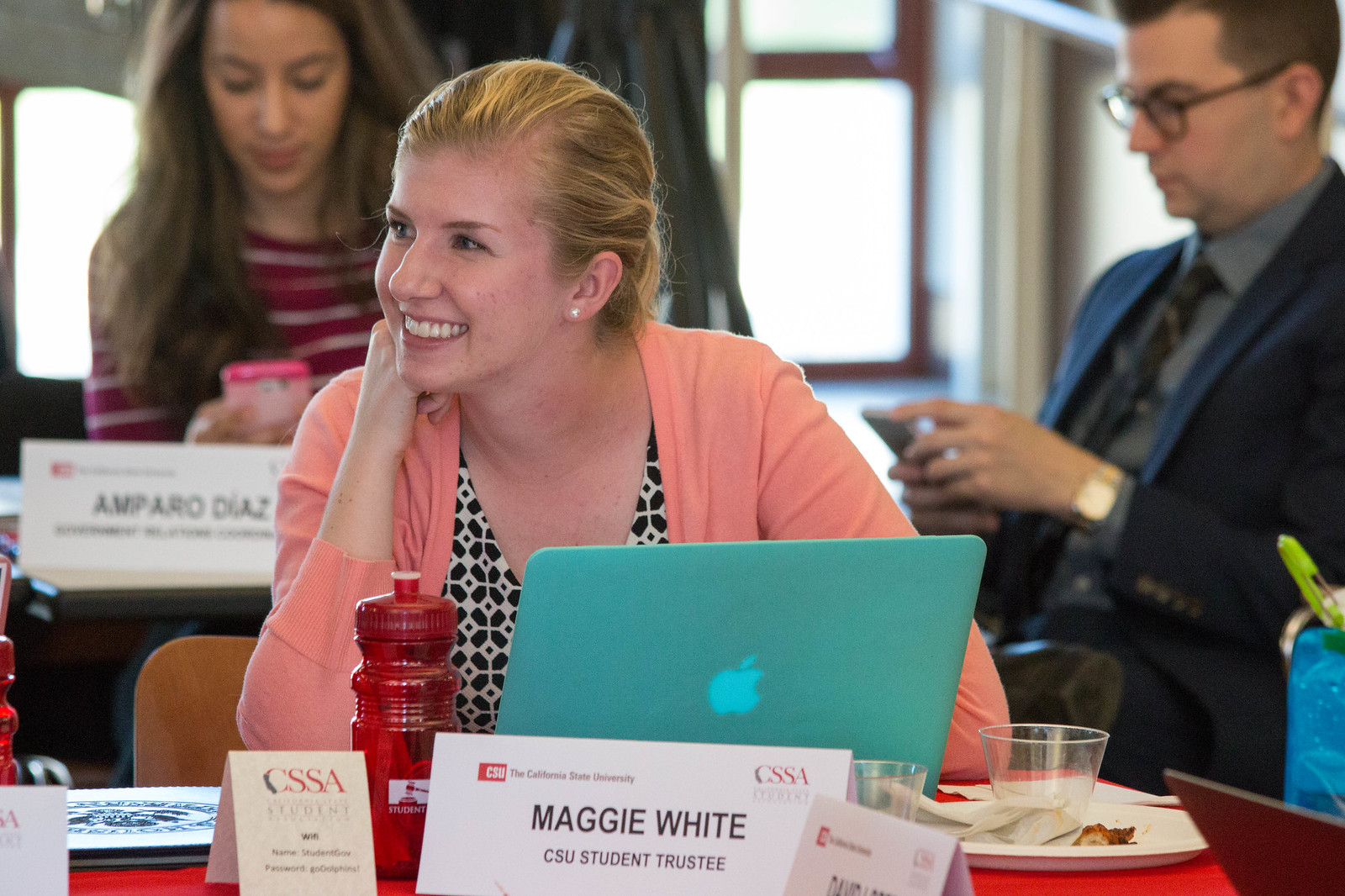A young Caucasian woman, Maggie White, is the focal point of the image, seated behind a table adorned with a red tablecloth, smiling broadly and looking to the left, revealing her top row of teeth. Maggie has brown eyes and her blonde hair is pulled back, complemented by ear studs. She is dressed in a pink sweater over a black and white patterned shirt. Her left arm rests below her chin, while her right arm is on the table behind a light green Macintosh computer with the Apple logo visible.

On the table, along with the laptop, there are several items including a red water bottle, a plate with some food, and various cards and signs. Prominently in front of her is a nameplate reading "Maggie White, CSU Student Trustee," displaying logos of CSU and CSSA, and another card indicating "Wi-Fi name and password."

In the slightly blurred background, a young woman with long blonde hair cascading over her shoulder is visible on the left, dressed in a red shirt with white stripes. She is engrossed in her white cell phone. On the right side of the image, a clean-shaven man with short hair and glasses is seen wearing a navy blue blazer, gray shirt, and black tie, accessorized with a gold wristwatch. He is also absorbed in his phone. The setting appears to be an indoor meeting or conference, accentuated by large glass windows with brown borders and white-gray walls in the background.